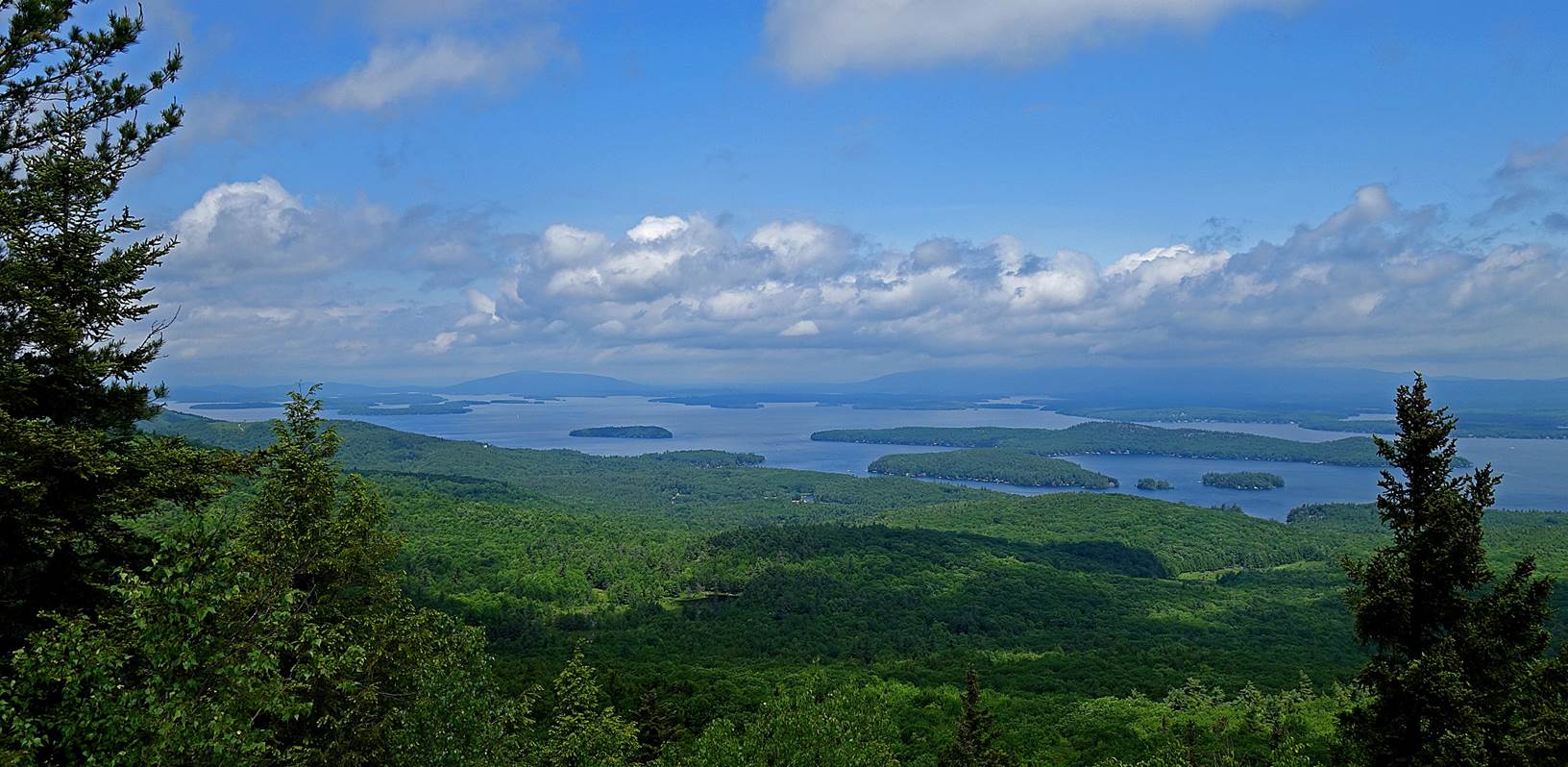In this realistic daytime photograph, a serene forest scene is depicted with a light gray sky softly illuminating the surroundings. The setting features an array of tall, green trees with brown trunks, complemented by an abundance of green bushes and patches of grass interspersed with brown dirt. Central to the image is an impressive and intricate statue of a meditating man, carved from wood, positioned atop a modest hill created by a group of large gray rocks. This statue stands about 10 to 15 feet tall and spans roughly 20 feet in width. The figure is cross-legged, with large hands resting gently to his sides, eyes closed, and mouth open, suggesting a tranquil state of meditation. The statue's layered wooden construction gives it a shingled appearance, and fine details include a shirt, large ears, and a small nose. The earthy tones of the statue and rocks contrast with the lush greenery and scattered fallen branches in the background, emphasizing the natural beauty and tranquility of the forest backdrop.